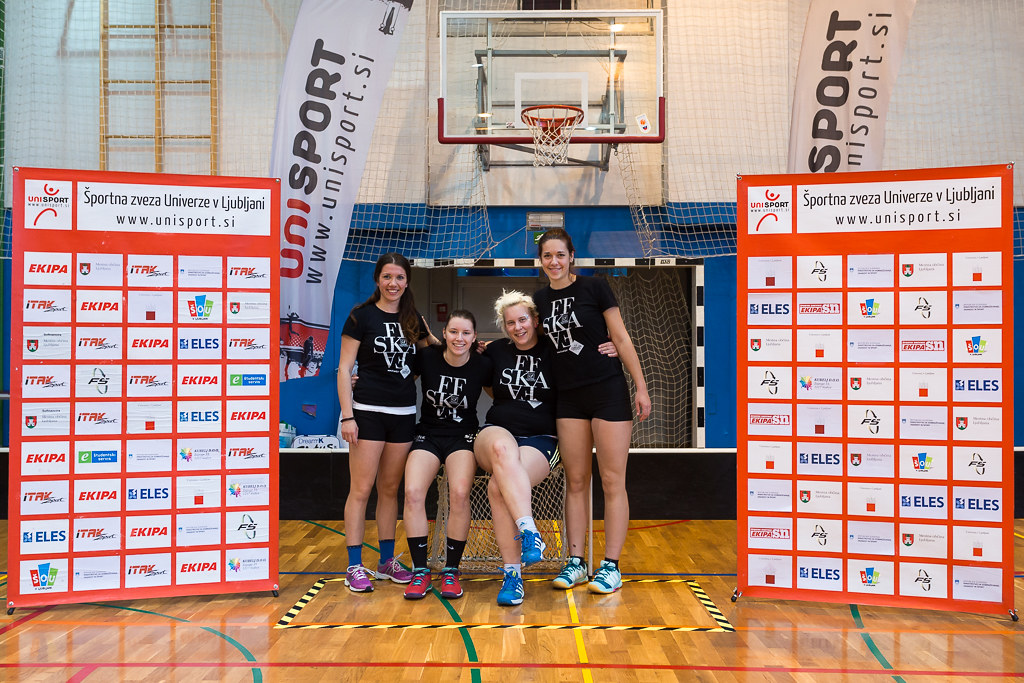In this detailed image, we see four girls positioned at the center of a polished hardwood basketball court, smiling directly at the camera. Two of the girls are seated in the middle while the other two stand on either side of them. Behind them, there's a basketball hoop and backboard, indicating an indoor gymnasium setting, most likely within a school and during the day. Flanking the group of girls on both sides are two orange signs on wheels. These signs display rows and columns of white squares that appear to contain logos, and at the top, they read "SPORTNA ZVEZA UNIVERZE VLJUBLI JANI". The scene is rich with vibrant colors, including brown, red, orange, green, yellow, black, purple, and pink, though all text appears to be in a different language.